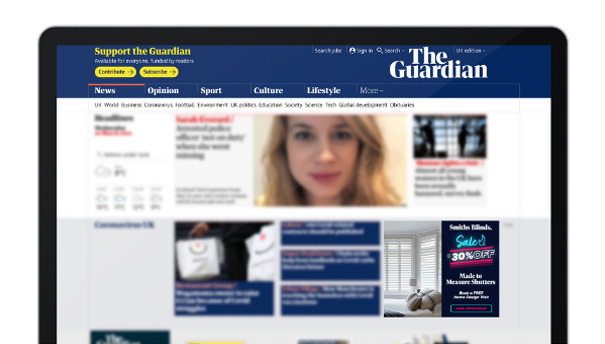The image appears to depict a laptop screen with a distinctly black bezel framing the display. The screen itself shows a web page distinguished by a blue header on the left-hand side containing yellow text that reads "Support the Guardian." Beneath this header is a section with indiscernible white text. Additionally, two clickable links are visible, denoted by blue text, each accompanied by a right-pointing arrow, though their specific content is unclear.

On the right-hand side of the header, white text prominently displays options that appear to say "Search jobs," "Sign in," then "Search." Above this section, the word "Guardian" is clearly written. Another portion of this header, consisting of white text, is present but illegible.

Below the header, the screen is divided into various interactive sections. On the left, five navigable buttons are arranged in the following order, each labeled with white text: "News," "Opinion," "Sport," "Culture," and "Lifestyle." Adjacent to these is a gray button labeled "More," featuring a dropdown menu.

Further down the page, blurred text sections are intermingled with buttons that display white text on blue backgrounds. At the center of the display is a somewhat blurry image of a blonde woman, who is gazing directly at the camera.

The right-hand margin of the screen contains a discernible section with a black background featuring white text. Prominently positioned within this segment is a blue text reading "Sale," followed by an offer of "30% off" written in a bubble font style, with the rest of the text remaining blurred and unreadable.